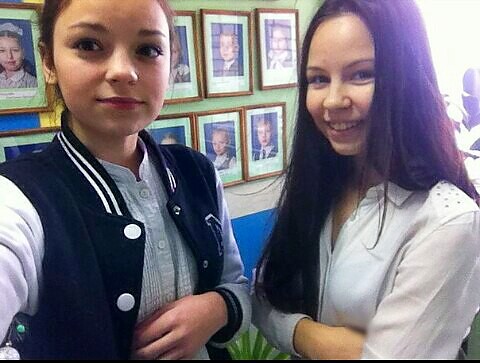This photograph captures two young women, likely in their late teens or early twenties, standing side by side in an office setting. The woman on the left is dressed in a high school-style starter jacket, featuring a dark blue body, white sleeves, and white stripes around the collar. Her jacket has an emblem that resembles an 'M,' though it's partially obscured. She pairs the jacket with a light blue blouse and has her hair tied back. Her left hand rests in front of her chest, while her right hand reaches for something out of the frame. The woman on the right sports long, dark brown hair that cascades well below her lower back and over her right shoulder. She is dressed in a white button-down shirt with long sleeves and stands with her arms crossed, smiling slightly. In the background, the green wall is adorned with numerous brown-framed photographs depicting children, both boys and girls, and there is a window letting in sunlight behind the woman on the right. A small green plant is visible between the two women, adding a touch of nature to the indoor scene.